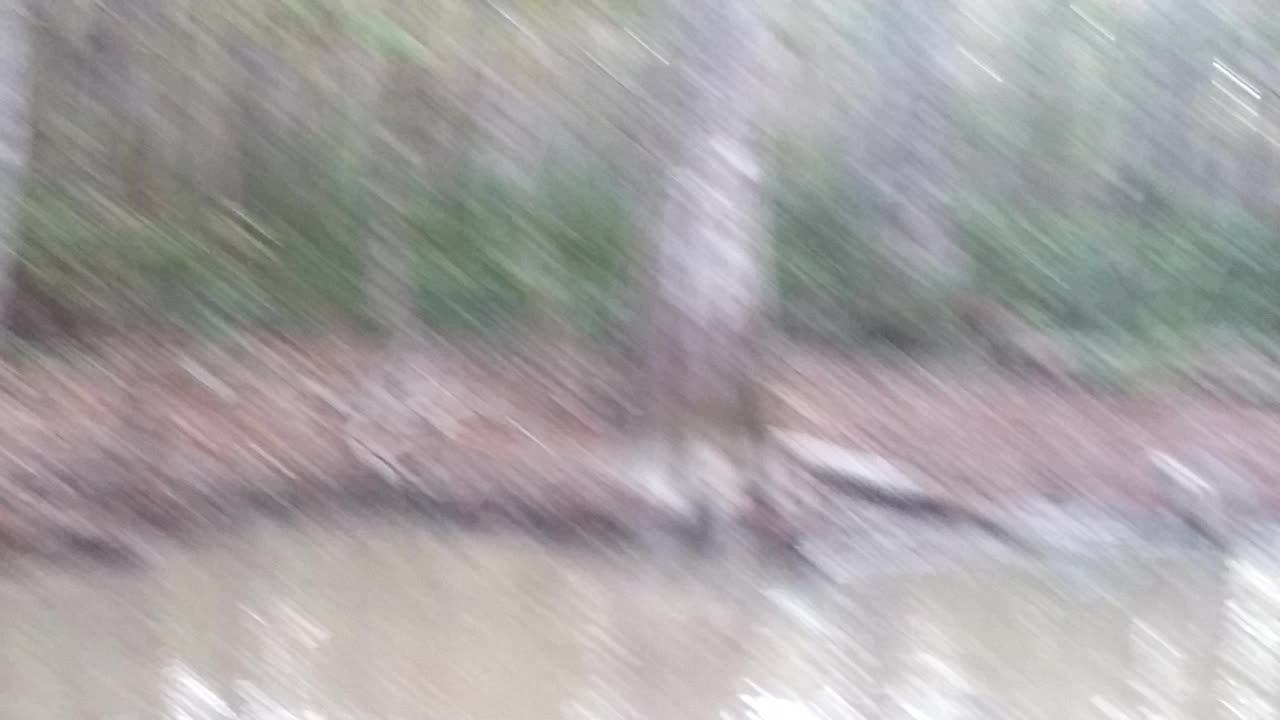Captured outdoors, this photograph exhibits significant motion blur, suggesting the camera was in motion when taken. The lower portion of the image reveals a small body of water, likely a river or pond, with murky grayish-brown water. The far bank of the water body stands out with a reddish hue, while the surrounding area is interspersed with gray tree trunks and lush green vegetation. Striations caused by the camera's movement streak diagonally from the top left to the bottom right, adding an abstract element to the scene. Scattered across the bank, a mix of logs and debris further enhances the rugged, natural setting.